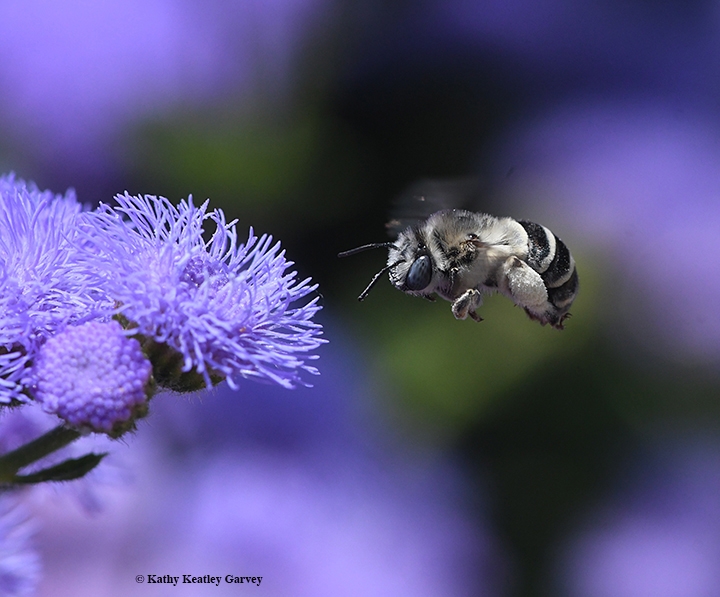This professional photograph by Kathy Keatley Garvey captures an extreme close-up of a bee, prominently positioned next to a violet flower. The bee, which resembles a honeybee but with distinct white and black stripes rather than the typical yellow and black, is detailed with a white furry abdomen and legs that appear to be dusted with pollen. The insect's large eyes are especially noticeable, although its wings are almost invisible due to their rapid movement as it flies toward the flower. The background is artfully blurred, highlighting the bee and flower while presenting a mix of muted colors, including yellow, dark tones, and purple hues. The entire scene exudes a sense of movement and natural beauty, with the bee diligently working against a backdrop that gives the impression of being illuminated by ultraviolet light. This image not only captures the essence of the bee's industrious nature but also emphasizes its aesthetic charm, adding a touch of personality and vibrancy to the otherwise subtle and ethereal composition. The photograph is copyrighted by Kathy Keatley Garvey, as noted in the bottom left corner.